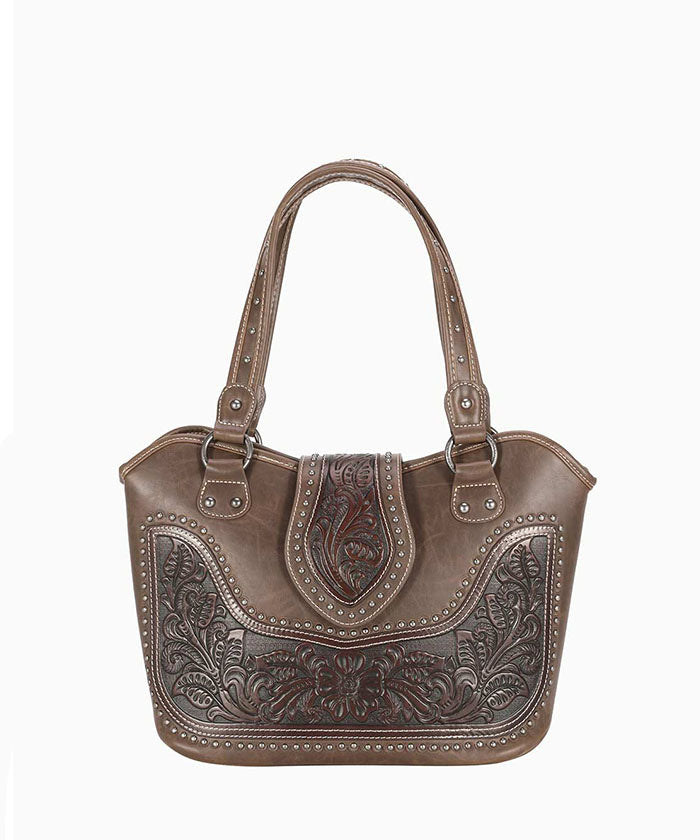This close-up photograph depicts a brown leather handbag with a detailed, intricate design. The bag, set against a white background, features leather straps standing straight up from the top and affixed at two points. The main body of the handbag is a rich brown, while a darker brown leather flap at the center adds a contrasting element. This flap, which secures the bag, is adorned with delicate embroidery, showcasing a flower motif surrounded by fleur-de-lis and leafy patterns. Small brass rivets accentuate the intricate designs on the darker leather, evoking a style reminiscent of cowboy boots. The bag also has a sturdy strap that can be used to carry it over the shoulder. The handbag is of a decent size, emphasizing both functionality and a touch of elegance through its detailed craftsmanship.